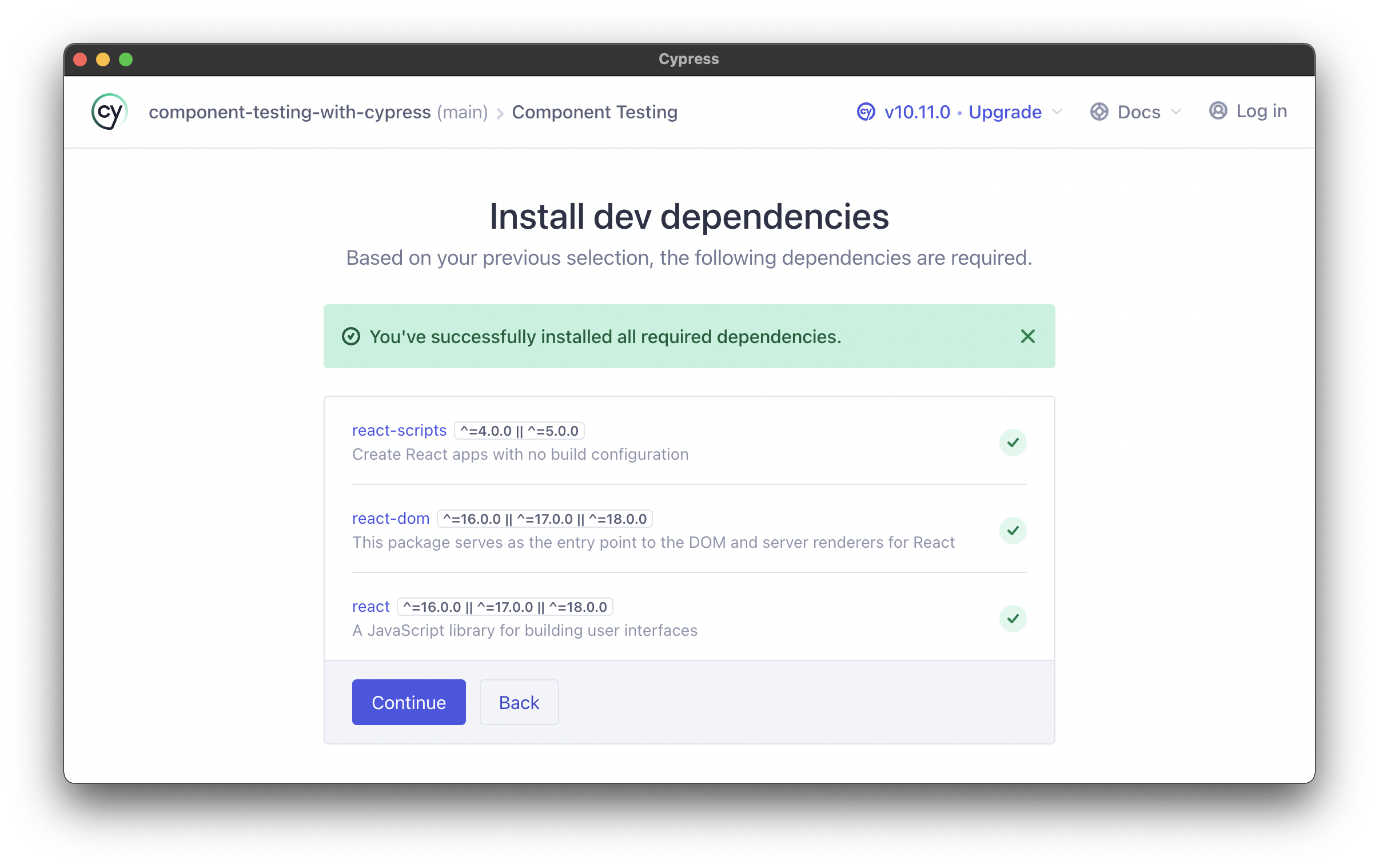The screenshot displays a partial web page from the Cypress website. At the top, there's a black banner featuring a series of red, yellow, and green dots, reminiscent of a traffic light. The Cypress logo, a stylized "CY" within a circle, is located to the right of this banner.

The page prominently displays the title "Component Testing with Cypress," with the subtitle "Main Component Testing." To the right, it shows the text "v10.11.0 upgrade" accompanied by a dropdown arrow, followed by quick links to "Docs" and a login icon.

Below this header, in a combination of black and white text, a section reads: "Install Dev Dependencies. Based on your previous selection, the following dependencies are required." 

This is immediately followed by a series of vertically ordered boxes containing green checkmarks:
1. A green box reads, "You've successfully installed all required dependencies," with a closeout 'X' symbol for dismissal.
2. "React Scripts: Create React apps with no build configuration," alongside a green checkmark.
3. "React DOM: This package serves as the entry point to the DOM and server renders for React," with another green checkmark.
4. "React: A JavaScript library for building user interfaces," also marked with a green check.

Towards the bottom, there's a gray box containing two buttons: a blue "Continue" button and a gray "Back" button.